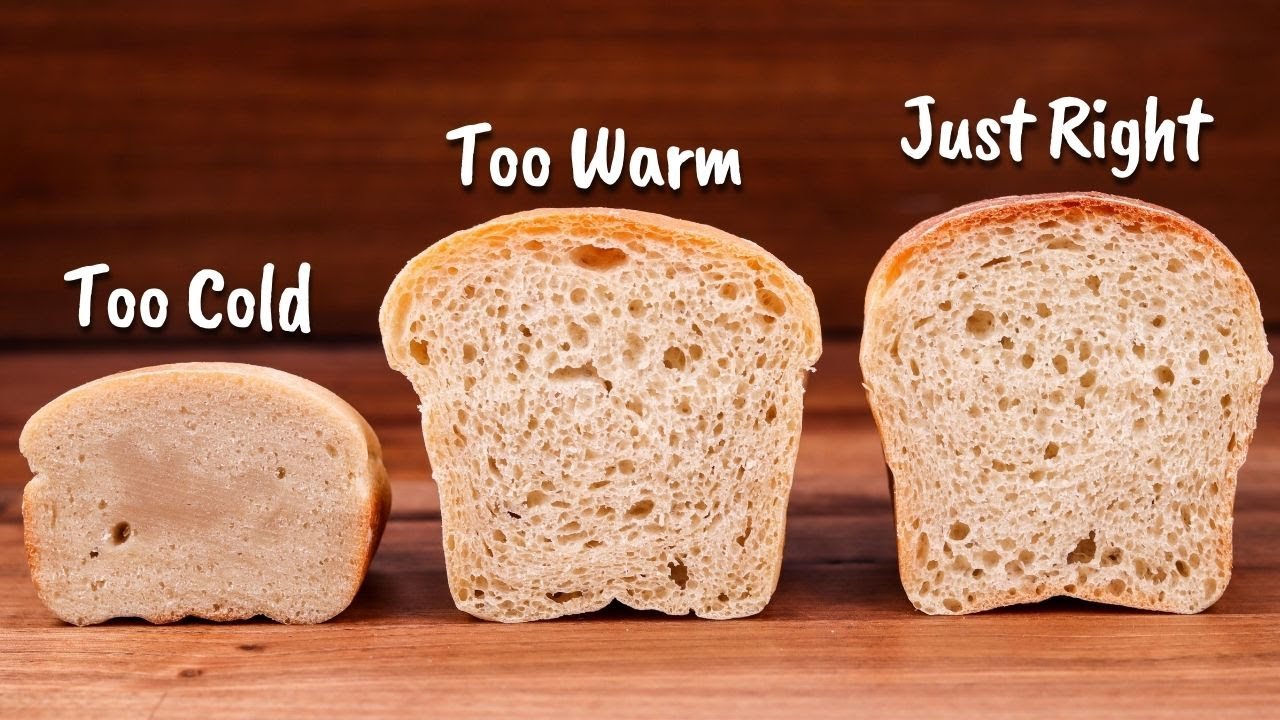The image depicts three slices of bread standing upright on a wooden table, aligned from left to right. Each slice is labeled with white text indicating its baking condition: "TOO COLD" on the left, "TOO WARM" in the middle, and "JUST RIGHT" on the right. The slice on the left, marked "TOO COLD," is noticeably smaller and denser, lacking fermentation air bubbles, and has a raw appearance in the center, perhaps resembling a undercooked loaf or even spam. The middle slice, tagged "TOO WARM," is larger and has visible air pockets indicative of fermentation, but appears overcooked. The slice on the right, labeled "JUST RIGHT," is the tallest, with a darker crust, and shows well-formed air pockets, suggesting a perfectly baked loaf. The photograph, which seems intended for a baking training manual, features a detailed wooden table grain and a similarly wooden background, reinforcing the rustic and handmade aesthetic.